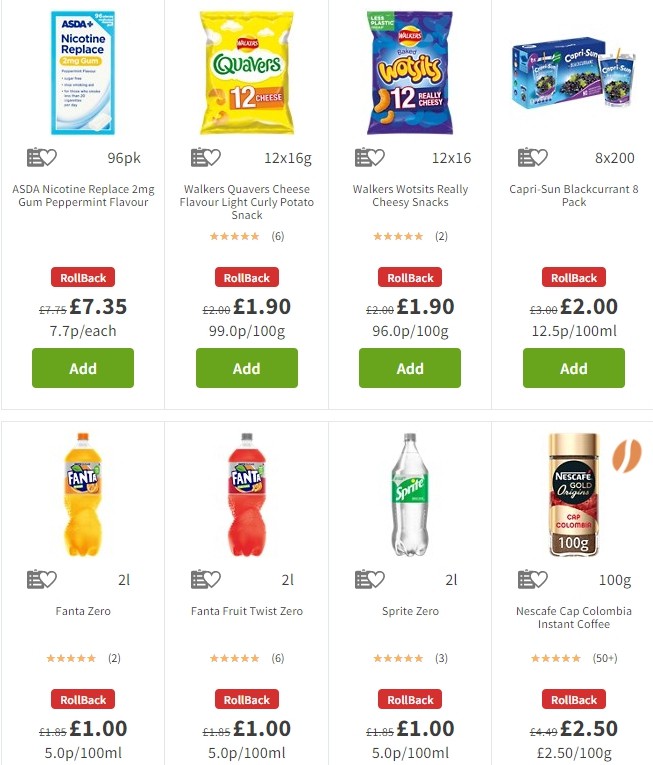This image is a detailed screenshot of a website showcasing a list of products. The background is entirely white, and each product is enclosed within a thin, light gray, vertically rectangular border. Each listing features a photograph of the product at the top, set against the same white background for uniformity. 

Below the photograph, on the left side, there is a dark gray clipboard icon, and adjacent to it on the right, a dark gray heart icon. Next to the heart icon, a package size is displayed. Moving further down, the product name is written in light gray text. Some products also display star ratings beneath the product name, with yellow stars indicating the rating and a number in parentheses in light gray text showing the number of reviews.

Each listing includes a red badge beneath the star ratings, with the word "rollback" written in white text, indicating a discount or price reduction. Below this badge, a previous price, shown in pounds, is crossed out in small gray text. To the right of this, the new price is prominently displayed in large, bolded black text. Another piece of information, showing the price per count or weight, is presented in medium-sized, medium gray text underneath the new price.

At the bottom of each listing is a green button with white text that says "add," allowing users to easily add the product to their cart.

The products are arranged in four columns per row and include the following titles:

1. ASDA Nicotine Replacement 2mg Gum Peppermint Flavor
2. Walker's Quavers Cheese Flavor Light Curly Potato Snack
3. Walker's Wotsits Really Cheesy Snacks
4. Capri Sun Black Currant 8-Pack
5. Fanta Zero
6. Fanta Fruit Twist Zero
7. Sprite Zero
8. Nescafe Cap Colombia Instant Coffee

Each product is clearly displayed with all essential information to facilitate easy browsing and selection for the user.